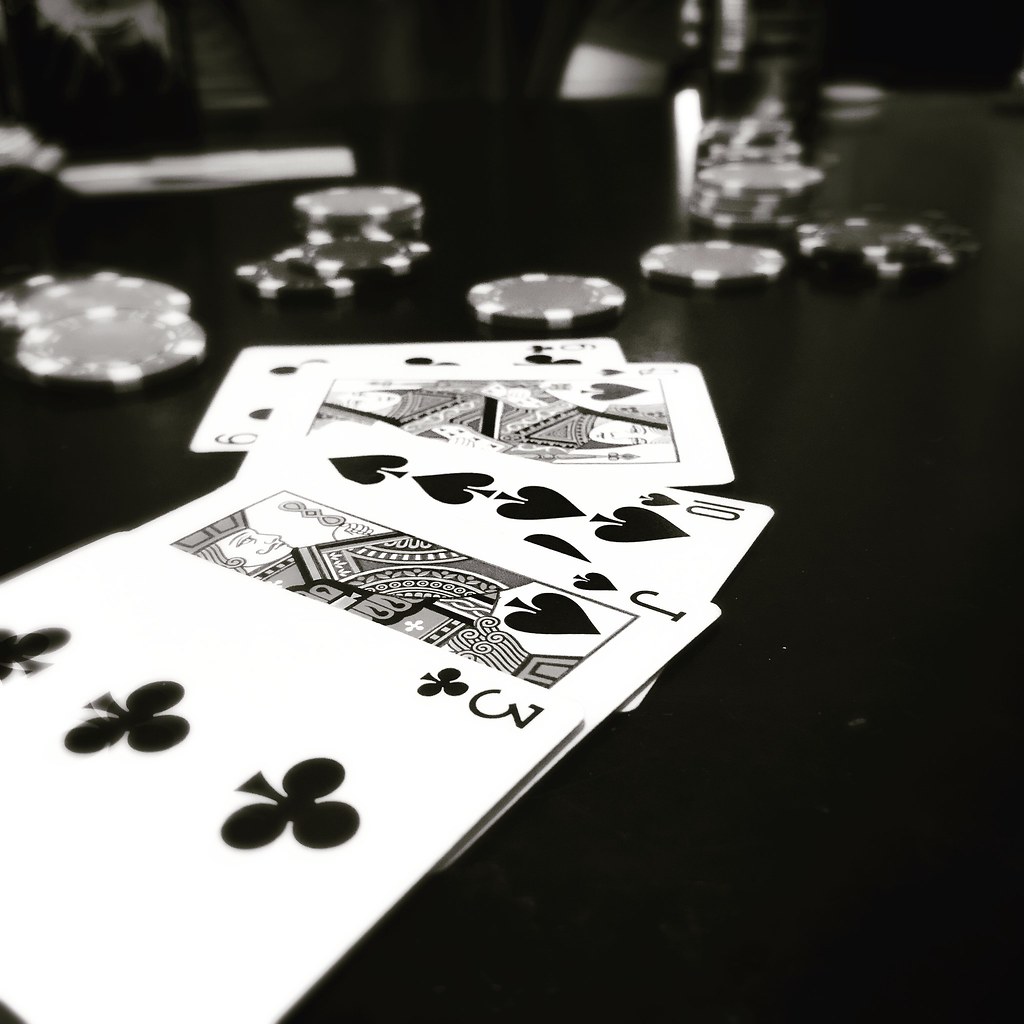This evocative black-and-white photograph captures an intense moment from a poker game. At the forefront, a large black table serves as the stage for this timeless scene. The main focus is on a spread of five playing cards, meticulously laid out in the center. Among the cards, you can clearly identify the three of clubs, jack of spades, ten of spades, queen of spades, and six of clubs.

Surrounding the cards are poker chips, scattered in various groupings across the table. To the left of the card spread, three chips lie in a small cluster, while another pile containing about six chips is nearby. Additional chips are dispersed with a hint of randomness: one stands alone, another pair hugs close together, and larger groupings of five or six are distributed around the players.

In the background, the scene is set against large, heavy curtains that add a sense of drama to the image. On the left side of the frame, an individual is partially visible, their presence hinted at by the edge of the table. To the right, another figure in a dark t-shirt is seated, with only their arm visible, partially obscured by the table. Near this person, there is a small stack of poker chips and what appears to be a drink, adding to the ambiance of the game.

In the back left corner of the table, additional cards or perhaps a piece of paper can be seen, suggesting ongoing strategies or potential hands still in play. The overall composition of this monochromatic image reflects the tension and focus often present in high-stakes poker games.